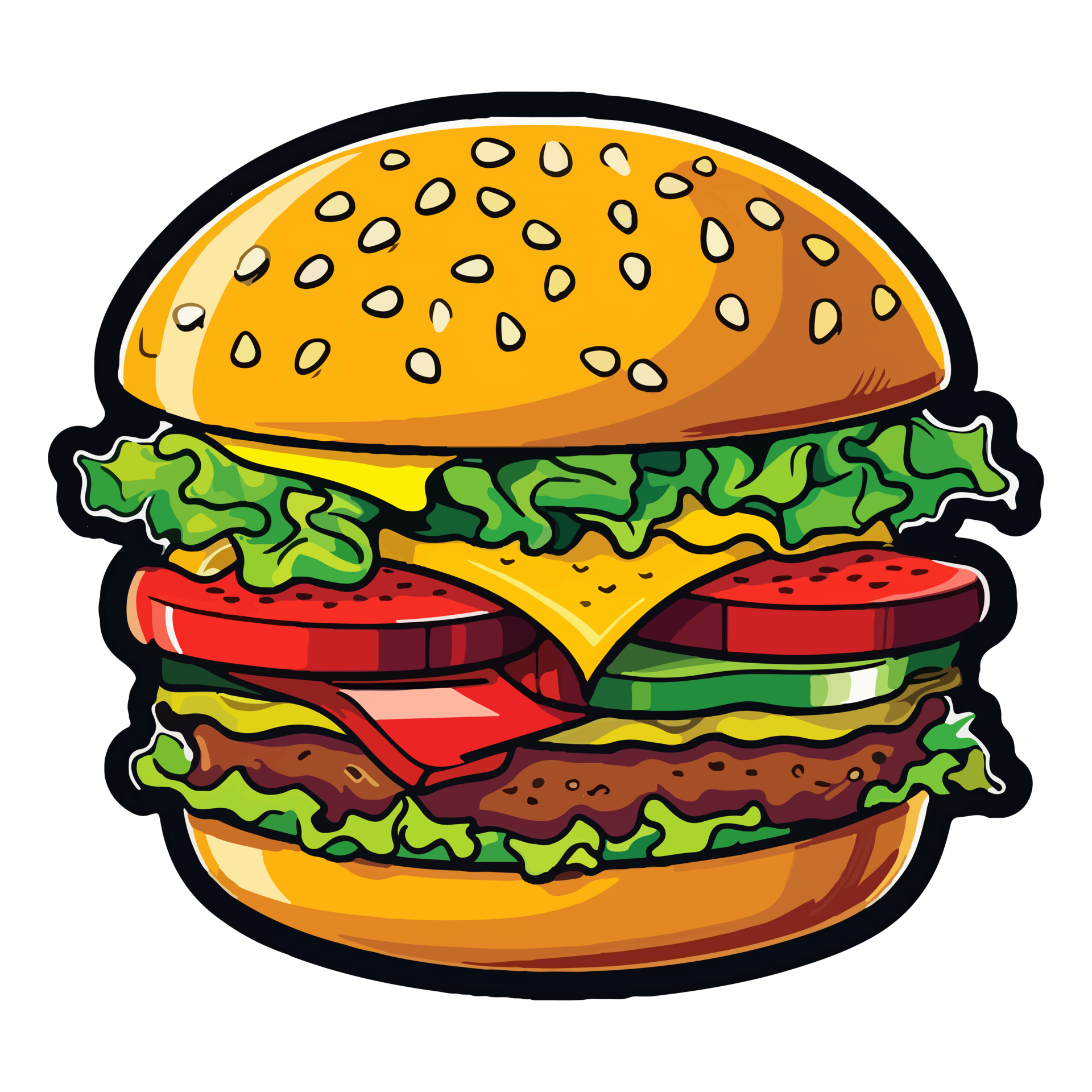The image features a vividly colored, highly stylized cartoon cheeseburger with a thick black outline. The cheeseburger has a visually striking combination of colors starting with a bright golden sesame seed bun on top. Below it, a sequence of layers is meticulously detailed: yellow-orange cheese, crisp green lettuce, another slice of yellow cheese, red tomato slices, green pickles, a strip of red bacon, and yet another slice of yellow cheese. All these ingredients rest atop a brown beef patty, which indicates that it is a beef burger. Underneath the patty, there's another layer of green lettuce followed by a similar golden sesame seed bun on the bottom. The image is filled with vivid colors making the burger elements pop, and it maintains a thick black outline that enhances its cartoony aesthetic.